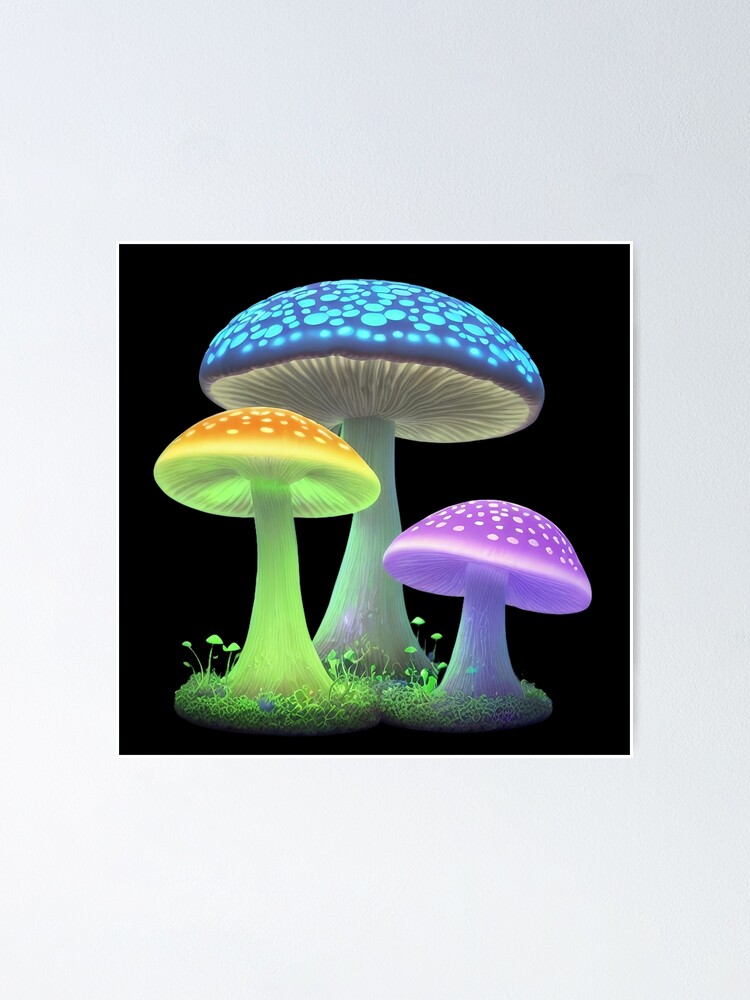In this digitally rendered image, set against a black square background with a larger gray border, three glowing mushrooms are prominently featured. The largest mushroom in the center has a striking neon blue cap adorned with light blue polka dots and emits a soft glow, resembling a luminescent lamp. Its stem is white, creating a vivid contrast. To the left, there's a mushroom with a fluorescent green stem that also lights up, coupled with a brown cap covered in white polka dots, giving it a unique lime-green glow. The right mushroom displays a purple cap with white dots, similarly emitting a radiant purple light. Below these mushrooms, small, crooked green shrubs can be seen, adding a natural touch to the scene. The entire composition, with its glowing mushrooms, intricate cap patterns, and gilled undersides, presents a fantastical and vibrant display on the dark backdrop.